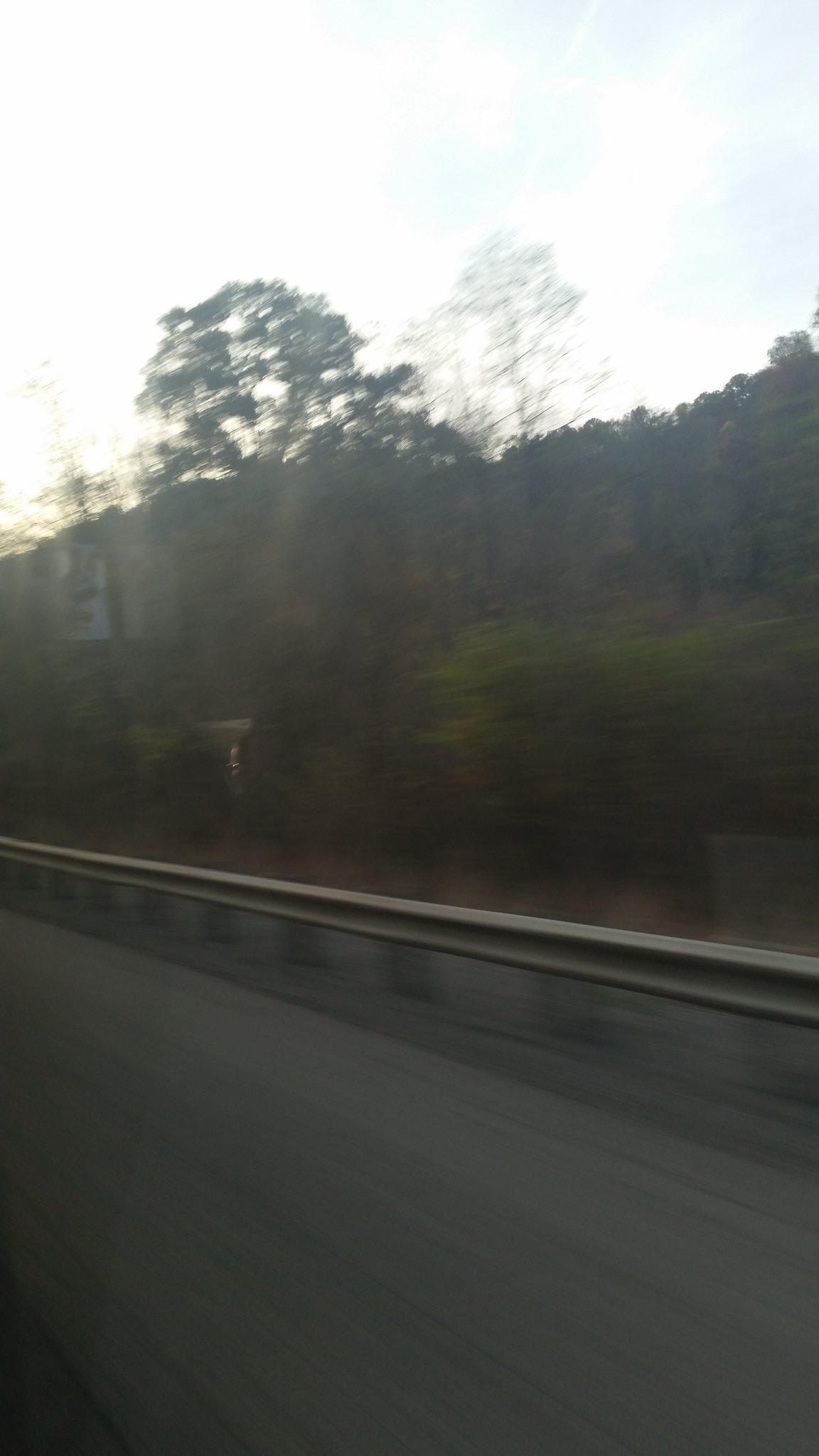This vertical, slightly blurry image, seemingly captured from a mobile phone, appears to have been taken from a moving vehicle. The motion blur suggests the vehicle was not traveling at high speed. The captured scene includes a partial view of a highway, characterized by a visible guardrail angled across the frame. Beyond the guardrail, a dense forested area is discernible, dominated by thick brush and several trees. One prominent tree stands out, extending over the surrounding foliage. The photograph, taken during the daytime, depicts the natural landscape and roadside elements in a candid, in-motion snapshot.